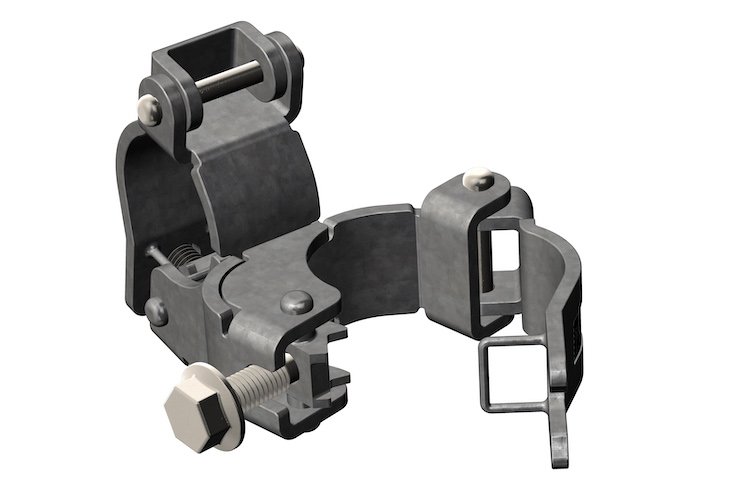The image depicts a detailed 3D rendering of a heavy-duty, dark gray mechanical clamp or bracket made of metal, set against a solid white background. The bracket features a prominent screw on the lower left side, which is light silver in color and currently untightened. This screw appears to be designed to lock a ring enclosure shut when turned. 

On the lower right side, the bracket has a latch mechanism that latches over to the left, with the untightened screw facilitating the latch's secure closure. The upper left section of the bracket is taller and features a horizontal silver bar between two round metal sections, along with a large cutout in the center revealing screw grooves. 

Towards the back, there is a mount with a spring mechanism, possibly for added tension, and bolts that likely allow the bracket to be attached to another surface or structure. The overall design suggests that it functions as a clamp to hold objects securely when the screw is tightened.